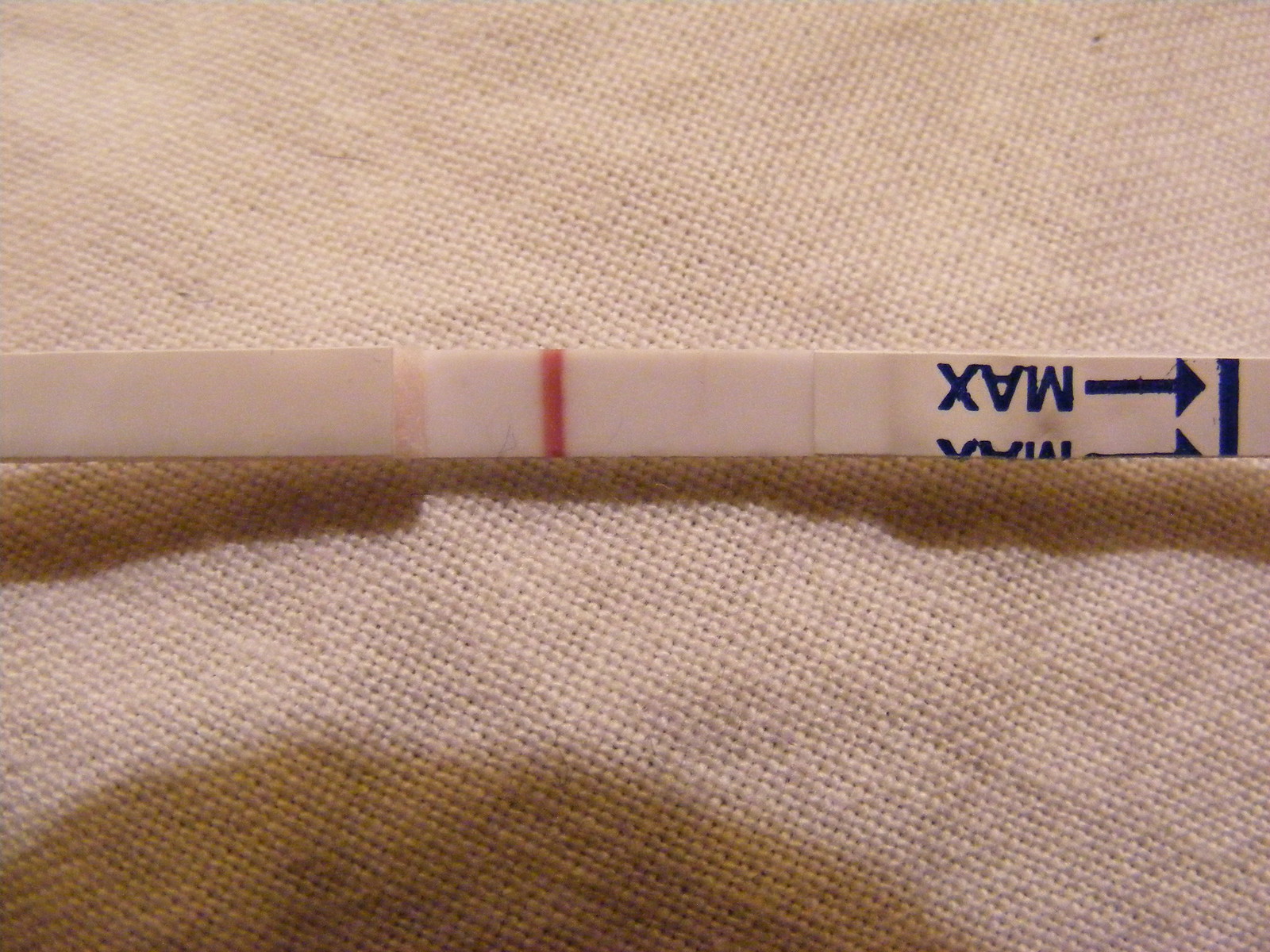The photograph, which is wider than it is tall, features a background of textured burlap material with a noticeable weave pattern. A subtle shadow appears at the bottom left-hand side of the image. The main focus is on a thin plastic strip positioned slightly above the midline, running parallel to the top and bottom edges of the photograph.

This plastic strip, likely a test of some sort, is marked with distinct features: a red vertical line, located just left of the center, and a blue vertical line. To the right of the red line, the word "Max" is written twice in blue, upside down. Accompanying this text is a blue arrow pointing to the right, followed by a blue band. The overall impression is that this strip measures something between the red and blue lines, with "Max" indicating a maximum threshold. However, the exact significance of the red line remains unclear.